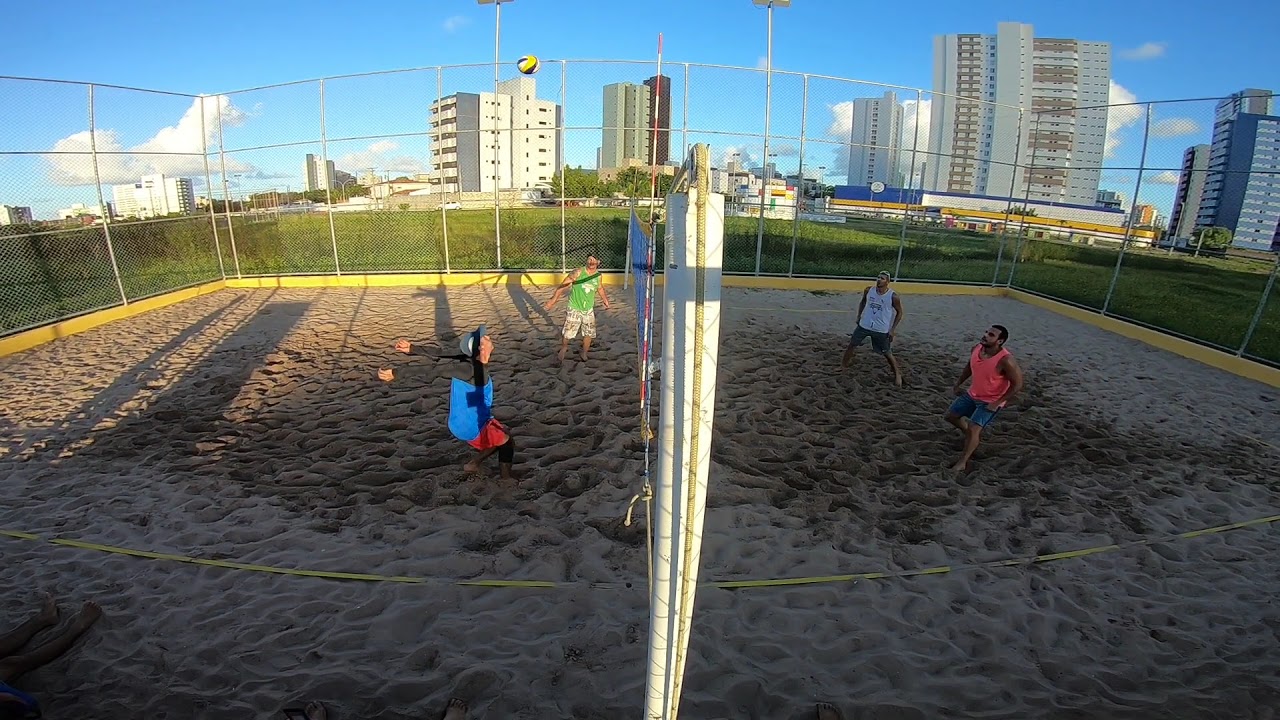In this horizontally aligned rectangular photograph, an outdoor beach volleyball game unfolds under a bright blue sky with a few fluffy white clouds. The beach volleyball court is enclosed by a very tall chain-link fence, and beyond this barrier, a vibrant green grass surrounds the area. The background reveals a city skyline adorned with multi-story buildings, predominantly beige with numerous windows, adding an urban charm to the scene.

On the sandy court, two teams of two male players face each other. On one side of the net, a man in an orange tank top stands beside a teammate wearing a white tank top. Opposing them, a man in a green tank top is partnered with a player dressed in a black and blue shirt and red shorts, who is kneeling with his arms behind him. Above this player, a volleyball is suspended mid-air, suggesting he is poised either to leap and strike the ball or has just completed a hit. None of the players are wearing shoes, emphasizing the casual, beachy atmosphere of the game.